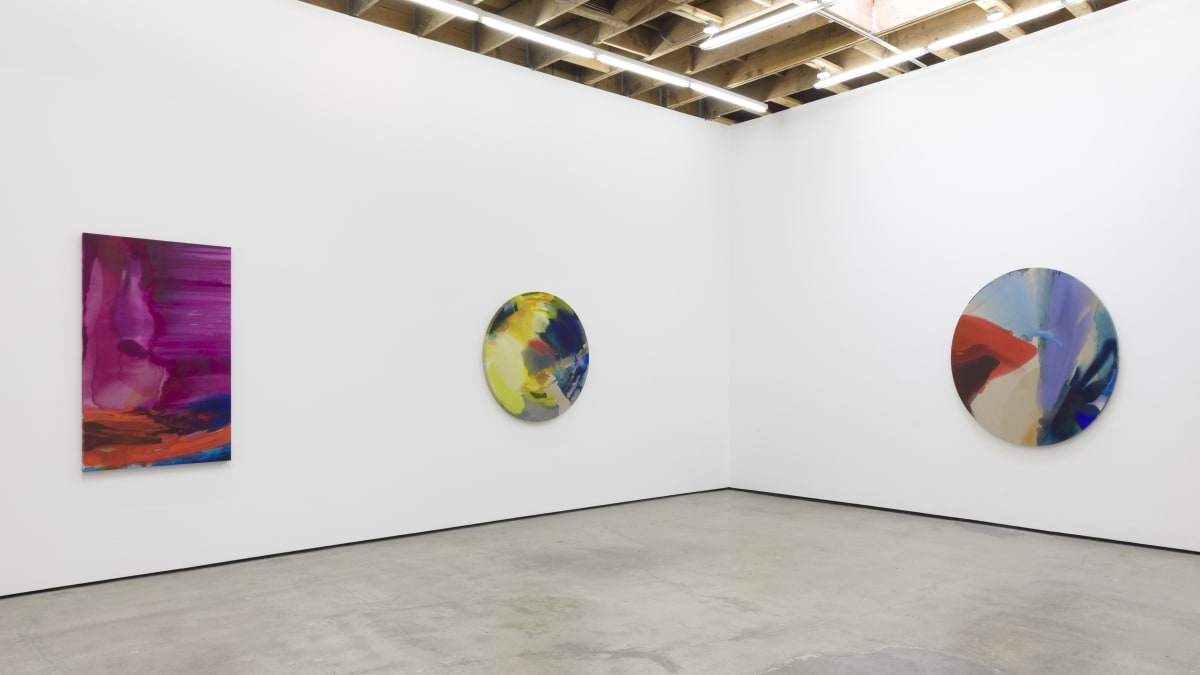The photograph displays an almost gallery-like room with a distinctly industrial ambiance. The white walls, unadorned except for three abstract paintings, contrast strikingly against the light-gray concrete floor. Two of the paintings are circular, while the third, situated more towards the left, is rectangular. The ceiling, an exposed grid of vents and lights, adds to the raw, warehouse-like atmosphere of the space. The rectangular painting is a vibrant mix of stripes and colors—pink, magenta, dark red, transitioning into blue and orange hues. The circular paintings feature a vivid palette as well, with the one in the middle suggesting a semblance of a female figure intertwined with blue, red, yellow, and gray swirls. The far-right painting maintains a similar colorful abstraction, blending white, blue, purple, and orange patterns. Each piece lacks descriptive labels, leaving their interpretation to the viewer's imagination. The room is otherwise empty, accentuating the stark and minimalist setting.